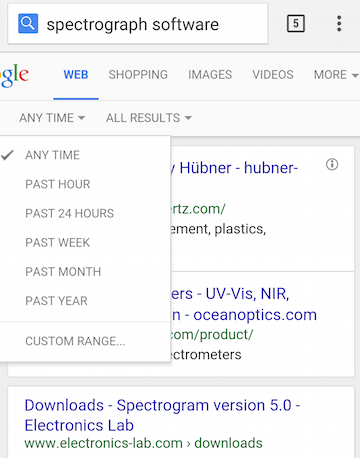The image is a vertically rectangular partial screenshot of a Google search results window. On the left side, the partial lettering "GLE" from the Google logo is visible, situated just above the search field containing the query "Spectrograph Software". To the right of the logo, the interface displays search options–Web, Shopping, Images, Videos, and more. The "Web" option is highlighted in blue with a corresponding blue underline.

Below these options are two drop-down menus labeled "Any Time" and "All Results". The "Any Time" menu is expanded, revealing its selections against a white background: "Any Time" (checked), "Past Hour", "Past 24 Hours", "Past Week", "Past Month", "Past Year", and "Custom Range". This expanded menu obscures parts of the first two search results. 

From the visible part of the search results, the far-right edges display text from the top two entries with the recognizable terms "Hubner" and "OceanOptics.com". The third search result, unobstructed by the menu, reads "Download Spectrogram v5.0 Electronics Lab".